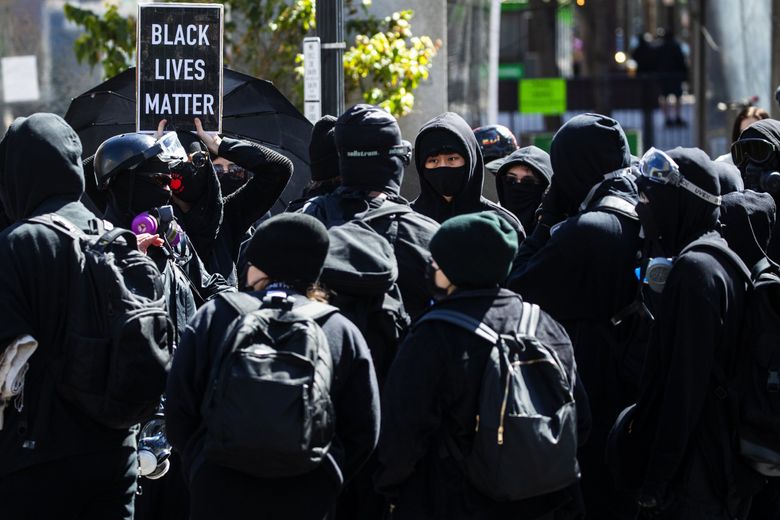This photograph captures a peaceful Black Lives Matter protest on a sunny day. A group of about a dozen people, dressed in black from head to toe—including hats, hoods, coats, and backpacks—are standing closely together outside in a city. Some of them are wearing additional protective gear like goggles and helmets, with one individual notable for wearing a purple gas mask. Near the center left of the image, a protester holds a black poster with a beige frame and white, center-justified text that reads "Black Lives Matter." Another protester beside them holds an open black umbrella. Though their faces are partially visible, revealing pale Caucasian skin, the protesters appear unified in their cause. The reflective sunlight illuminates the branches of a tree and highlights a building facade in the background, enhancing the overall peaceful and orderly atmosphere of the scene.